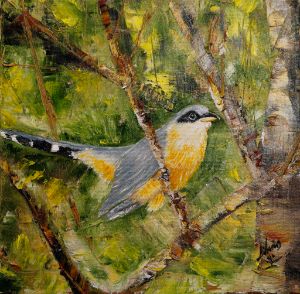This vibrant and detailed watercolor painting captures a colorful bird, possibly resembling a mockingbird or robin, perched on a branch in the heart of a large tree. The bird, positioned centrally and viewed from the side, showcases a vivid palette: its chest is a striking orange or reddish hue, while its wings and back transition between shades of gray and blue, accented by black-and-white stripes on its tail. The bird's eye is surrounded by a distinctive mask-like black area, giving an alert look as it gazes into the distance. The branch it perches on extends from the tree trunk, which is visible along the right side of the artwork and appears in mixed tones of gray and brown. The lush background is a lively collage of green and yellow splotches, representing foliage and leaves in various stages of brightness. Scattered among these tones are hints of orange and yellow on the branches and tree bark. A barely noticeable, cursive signature, likely the artist's, is found in black ink in the bottom right corner, blending subtly into the painting's dynamic color scheme.